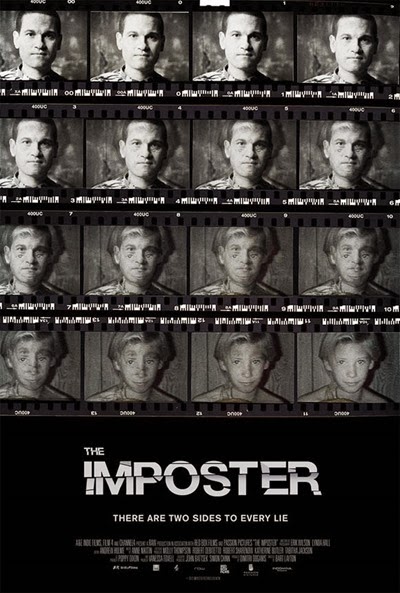This captivating movie poster for "The Impostor" features a unique and intriguing design centered around a series of film negatives arranged in a four-by-four grid. Each subsequent frame in the sequence reveals the gradual transformation of an adult man, Frederick Borden, into the young boy he is impersonating, Nicholas Barkley. The images progress from the top left corner, where the man with short, cropped brown hair is shown, to the bottom right corner, depicting a boy with longer, blondish hair, showcasing the striking metamorphosis across the grid. The entire sequence is presented in black and white, enhancing the dramatic effect. Below the film negative grid, the bold title "THE IMPOSTOR" is displayed in all caps, featuring a distinctive shatter effect that causes some letters to appear off-center and misaligned. Beneath the title, the tagline "There are two sides to every lie" is prominently displayed, adding to the mystery and tension of the film. The bottom section contains the standard movie credits, rendered in small, thin, all-caps lettering, supplemented by certain logos, completing the official and professional appearance of the poster.